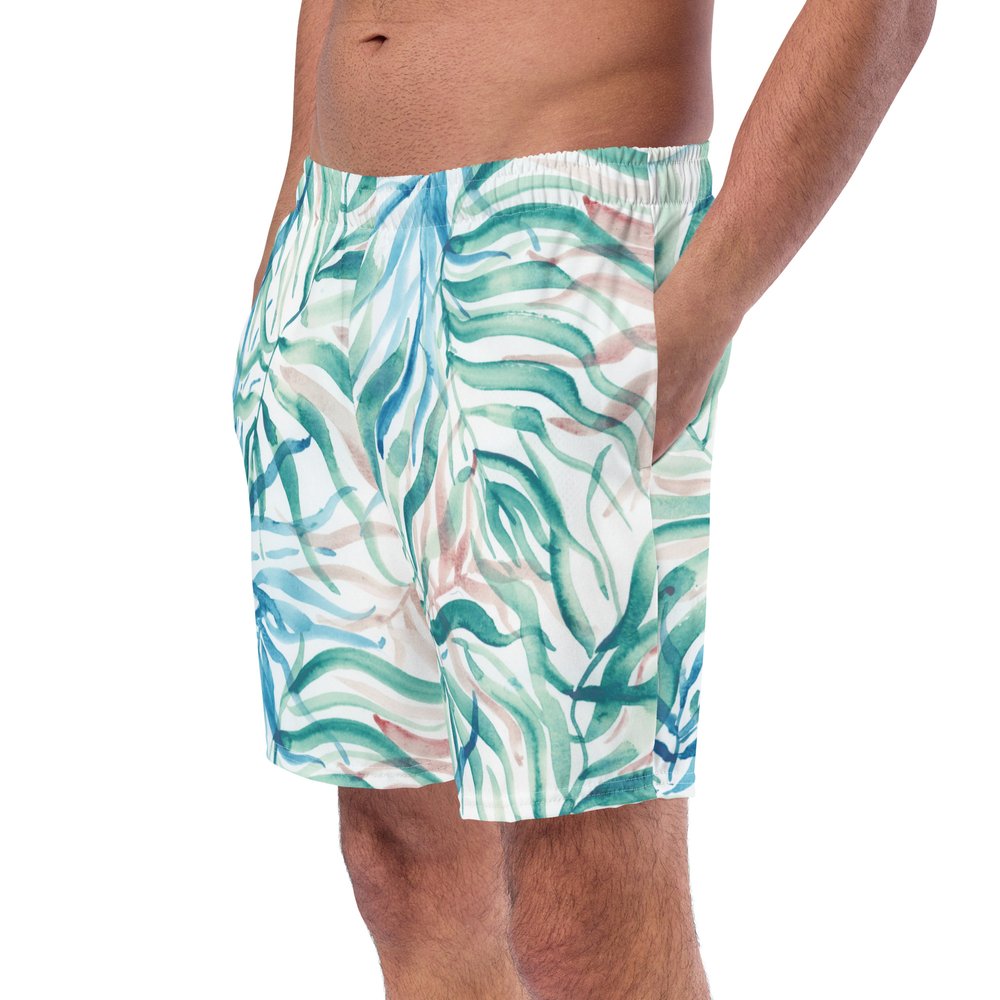In this catalog image from a clothing retailer's website, a fit male model is showcasing a pair of stylish swim trunks. The model is shown from just above his navel to just above his knees, with his left hand casually placed in the left pocket and a hint of his right hand suggesting it's in the right pocket. The swim trunks feature a cream base color adorned with a watercolor pattern of palm leaf fronds in wavy brush strokes of blue, green, and reddish hues, resembling abstract floral designs. The model's thin, slightly hairy legs and muscular build are clearly visible against the stark white background, which is evenly lit to eliminate any shadows and highlight the vibrant colors and details of the shorts. The swim trunks sit just below his navel and end just above his knees, perfectly suited for a summer look.